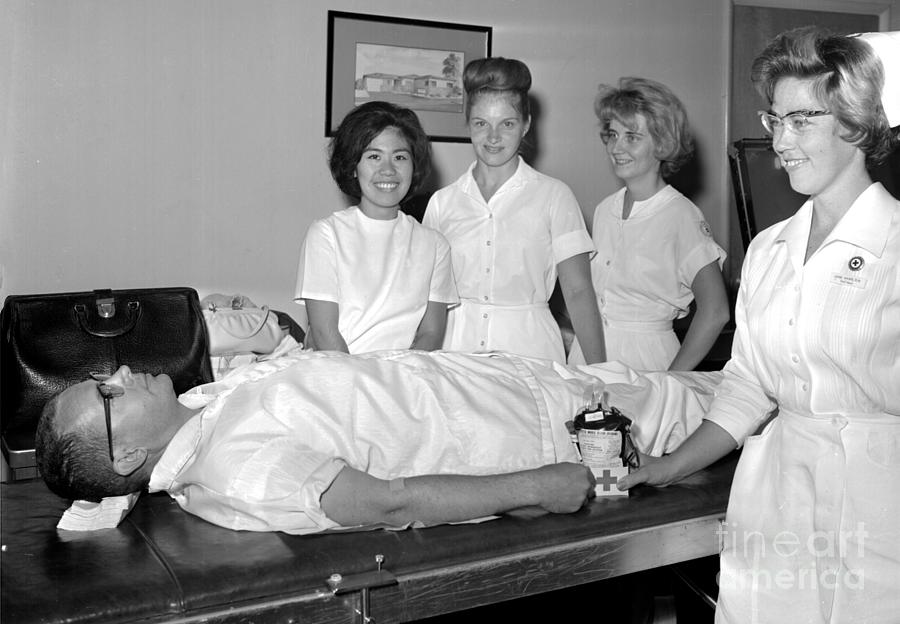This detailed black and white photograph, seemingly from the 1950s or early 1960s, depicts a medical scene involving a man dressed in white attire, suggesting he might be a doctor or nurse. He is lying on a metallic medical table, arms by his sides, and wearing black-framed glasses. Surrounding him are four women who appear to be nurses or medical staff, all dressed in traditional white uniforms.

In the foreground, a nurse stands to the man's right. She has curled back hair, cat's eye glasses, and wears a prominent 1950s nursing cap with a pin, indicating she might be an RN. She is holding onto a cart, which features a Red Cross symbol, possibly containing medical supplies.

Behind the man are three more nurses. The first of these is an Asian woman, and the two behind her are Caucasian. Two of the nurses, one with a bun and another with shaggy hair, are smiling and looking directly at the camera, while the remaining two are focused on the patient. The Asian nurse beside the man appears to be holding an oxygen or medical device, smiling. The man on the table also has a small bandage around his elbow, indicating recent medical attention.

In the background, there is an old school doctor's bag positioned near the man's head, along with a white bag. A framed drawing or picture of a building also hangs on the wall, serving as the sole piece of wall decor in this minimalistic and clinical setting. Overall, the ambient smiles of the nurses contrast with the man’s neutral expression, making the scene appear possibly staged or as a demo in a medical environment.